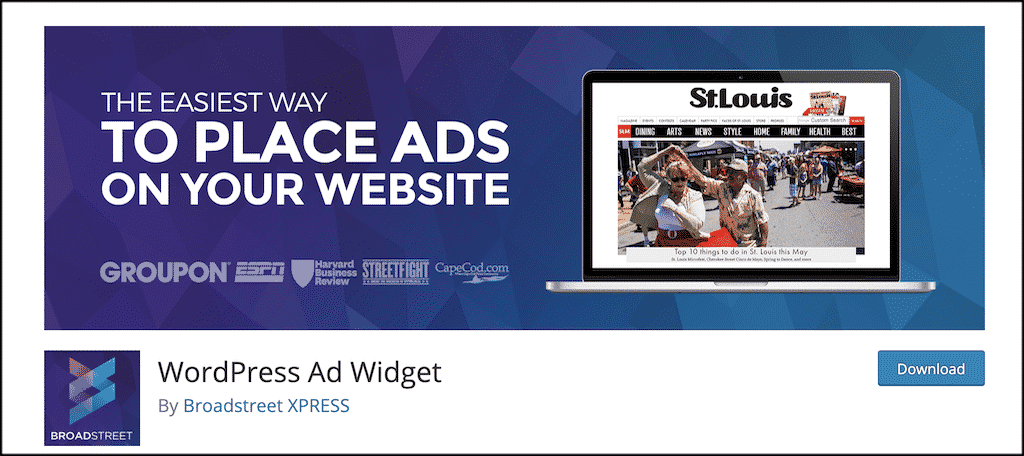The image features a clean, white background outlined in black, with a central, prominent blue box containing white text that reads, "The easiest way to place ads on your website." Below this message are logos and names of various notable entities, including Groupon (in purple), ESPN, Harvard Business Review, Street Fight, Caps Cake Custom, each accompanied by their respective icons.

On the right side of the image, there is a depiction of a computer screen framed in black, showcasing a white inner screen. The screen displays content related to St. Louis in black text, alongside a small newspaper icon. Beneath this, within a black box are various headings, with a central image of a man and woman amidst what appears to be a lively street carnival. The scene includes numerous people dancing in the street, lending a festive atmosphere to the depiction.

Separated by a large white line, the lower section of the image features a white background with a purple box containing the text "Broad Street" and decorative swirly lines that say, "WordPress ad widget by Broad Street Express." To the right of this text is a blue download button.